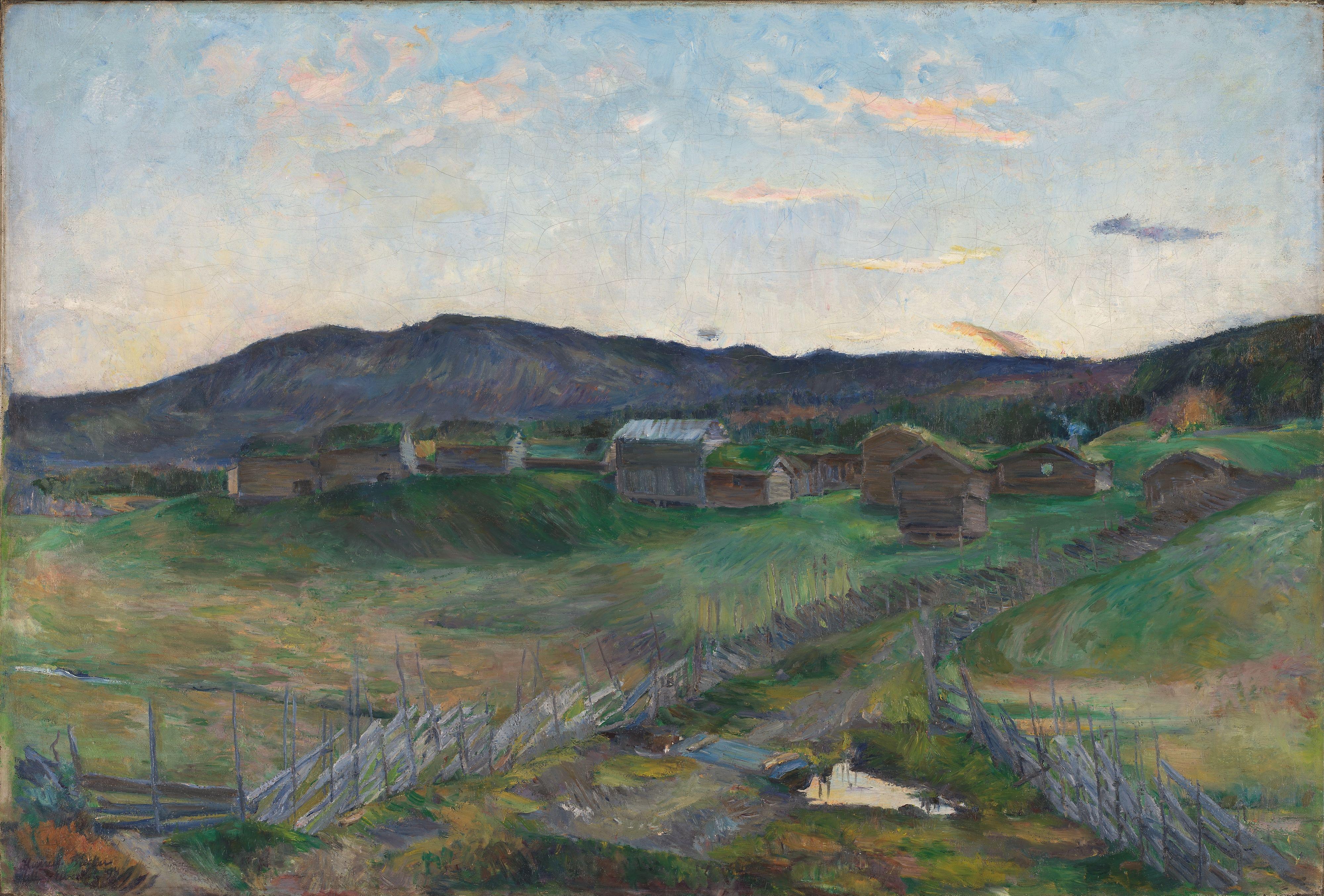The painting depicts a serene countryside scene that captures the tranquil charm of rural life. Dominating the foreground is a lush field of green, yellow, and brown grasses, gently blending into one another under the subtle play of light. Intersecting this field is a dirt road, partially overgrown, which curves gracefully from the bottom middle toward the top right. Flanking the road are two wooden fences that stretch back and to the right, converging near a small stream that pools into a reflective puddle. 

In the heart of the composition, spanning from left to right, stands a collection of over ten wooden buildings. These structures— a mix of sheds, barns, and farmhouses, some with gabled roofs and others thatched—are painted in earthy browns and whites, lending an authentic rustic feel to the scene. Behind these buildings, the landscape rises into a series of dark, blackish-brown mountains, adding a sense of depth and majesty.

The sky above is mostly clear, showcasing a soft blue canvas dotted with hints of yellow, white, and orange clouds, suggesting either early morning or late afternoon light. The sun itself is not visible, but its indirect rays illuminate the undersides of the clouds beautifully, creating a gentle, warm glow that enhances the overall idyllic atmosphere of the painting.